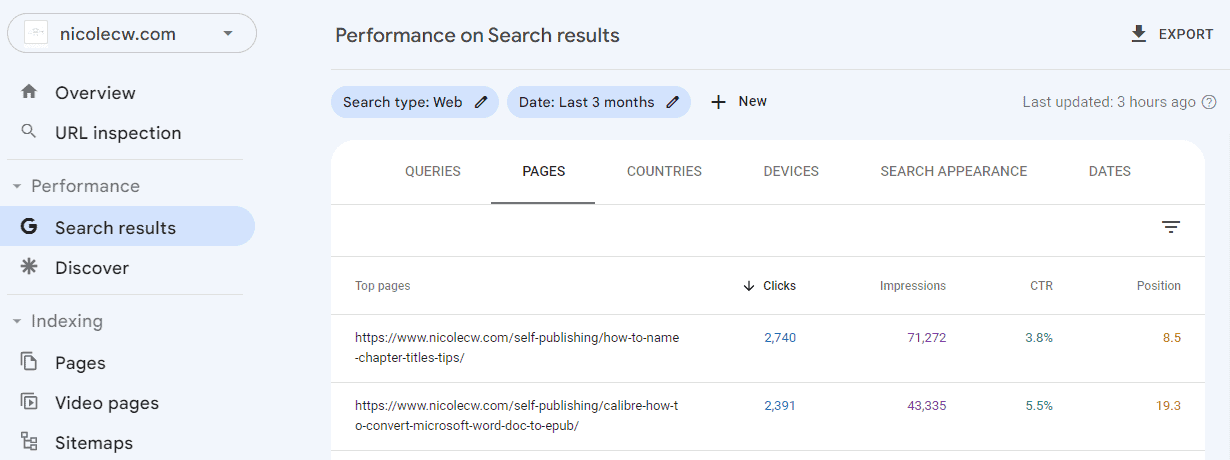This screenshot features a user interface on a predominantly white background framed by a light blue border. On the left side, the main focal point is an oblong, elliptical shape with the text "NicoleCW.com" inside. Below this, a menu begins with a home icon labeled "Overview." Adjacent icons include "Search" and "URL Inspection." Directly below these is the "Performance" drop-down menu, which further contains "G," "Search results," and an icon resembling a spiky star labeled "Discover." Following this, another drop-down menu titled "Indexing" lists options for "Pages," "Video pages," and "Sitemaps."

At the center of the screen, the first line prominently displays the text "Performance on Search results," followed by a rightward arrow icon adjacent to the term "Export." This section is immediately followed by three interactive elements: the first button labeled "Search type: Web" is blue, the second button saying "Date: Last three months" is also blue, and the third button, colored white, reads "+ New" and is intended for initiating a new tab.

Below these buttons, another section includes headings such as "Queries," "Pages," "Countries," "Places," "Search Appearance," and "Dates." 

Under these headings, a list is presented:
1. "Top Pages" accompanied by a count of clicks, showing URLs like "HTTPS://NicoleCW.com/self-publishing/house-name-chapter-titles-tips/"
2. Additional lines with similar URL structures.